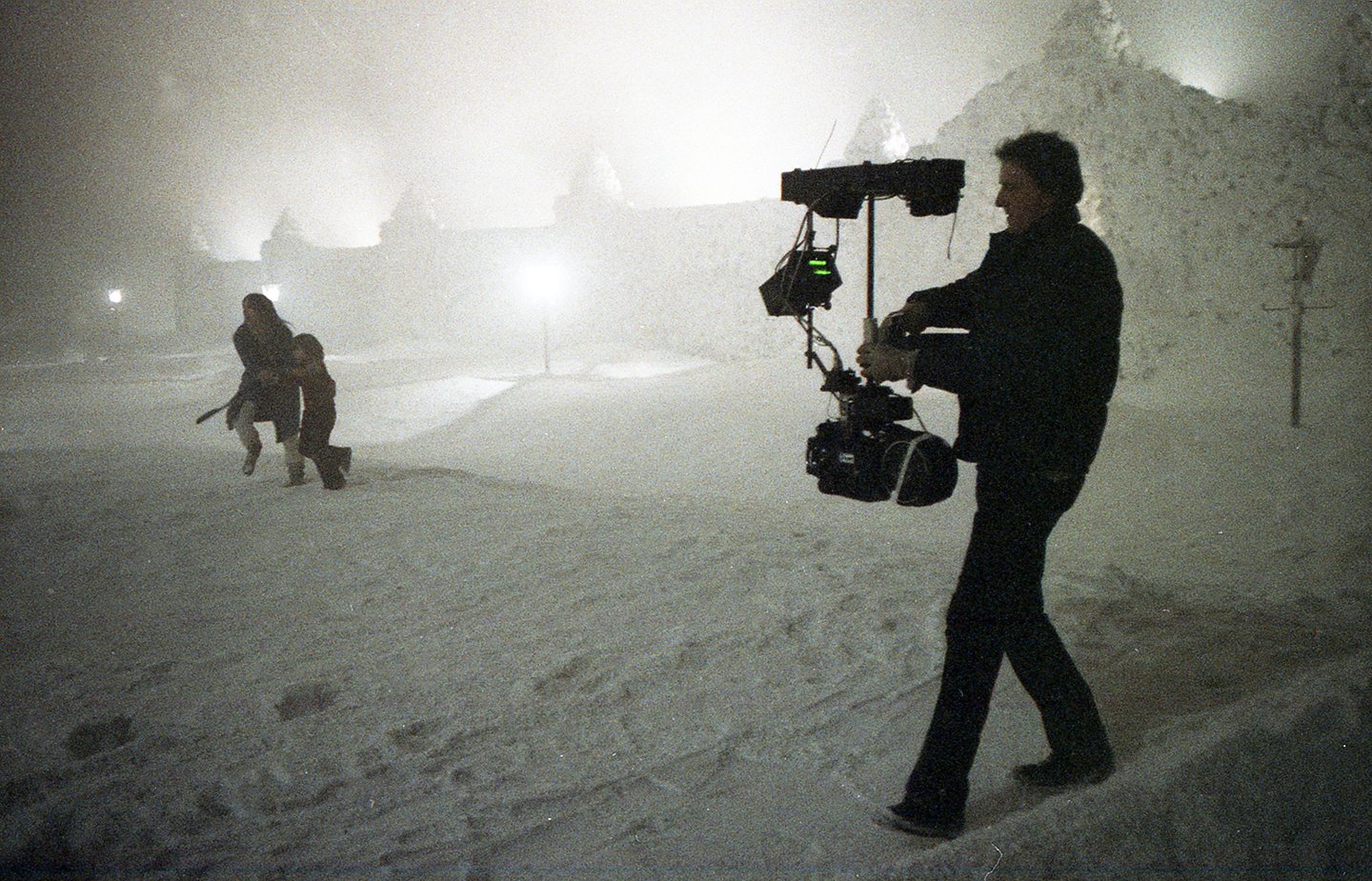The image depicts a horizontal rectangular movie set scene in the midst of a heavy snowstorm. Dominating the foreground on the right is a white male cameraman dressed in black, who is focused on filming with a complex camera setup, emitting a faint green light from one of its screens. The man is capturing footage of a woman and a child dressed in winter attire, with the woman in a black coat and white trousers. They appear to be running across the snow-covered ground, leaving tracks behind them. 

In the background, partially obscured by the falling snow and thick haze, are several buildings with a few lit windows, suggesting a town setting. Among these, five towers and a stone wall can be faintly discerned, further contributing to the scene's atmosphere. The visual narrative suggests a sense of urgency as the woman and child hurriedly move away from something unseen in the snowy landscape.